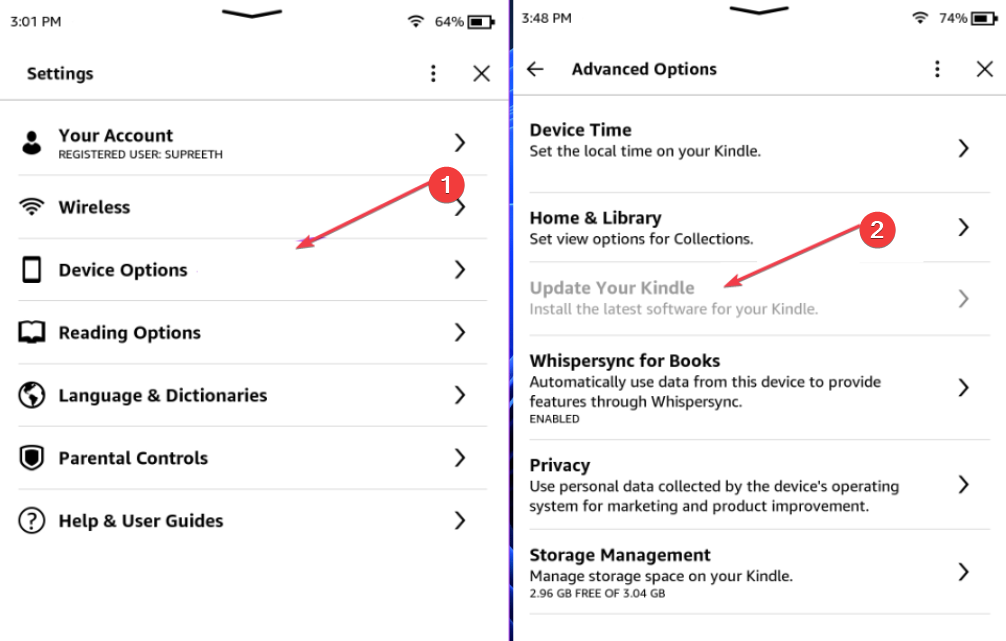The image depicts two screens on a Kindle device, each displaying different sections of the settings menu. The screens are separated by a distinctive blue and black vertical line. Both screens feature black headings on a pristine white background.

**Left Screen:**
- **Top Information:**
  - **Time:** 3:01 PM
  - **Battery:** 64%, represented by a battery symbol approximately two-thirds full.
- **Main Heading:** Settings
- **Additional Controls:**
  - Three vertical dots on the right for additional options.
  - An 'X' icon for deleting.
- **Categories:**
  1. **Your Account:** 
     - Icon: Torso and head outline
     - Label: Your account, Registered user: Supreet
  2. **Wireless:** 
     - Icon: Curved bars
  3. **Device Options:** 
     - Icon: Screen of a cell phone
     - Additional Indicator: Red arrow with '1' in a red circle
  4. **Reading Options:** 
     - Icon: Open book
  5. **Language and Dictionaries:** 
     - Icon: Globe
  6. **Parental Controls:** 
     - Icon: Shield with a black center
  7. **Help and User Guides:** 
     - Icon: Question mark in a circle
  - Each category label has a right-facing caret on the right side.

**Right Screen:**
- **Top Information:**
  - **Time:** 3:48 PM
  - **Battery:** 74%, with a corresponding symbol.
- **Main Heading:** Advanced Options
- **Additional Controls:**
  - Left-pointing arrow
  - Three vertical dots for more options
  - An 'X' icon for deleting
- **Categories:**
  1. **Device Time:** 
     - Description: Set the local time on your Kindle
  2. **Home and Library:** 
     - Description: Set view options for collections
  3. **Update Your Kindle:** 
     - Description: Install the latest software for your Kindle
     - Indicator: Red arrow with '2' in a circle
     - Status: Option grayed out (ghosted in gray font)
  4. **WhisperSync for Books:** 
     - Description: Automatically use data from the device to provide features through WhisperSync
     - Status: Enabled
  5. **Privacy:** 
     - Description: Use personal data collected by the device's operating system for marketing and product improvement
  6. **Storage Management:** 
     - Description: Manage storage space on your Kindle
     - Storage Status: 2.96 GB free of 3.04 GB

Each category label on this screen also features a right-facing caret.